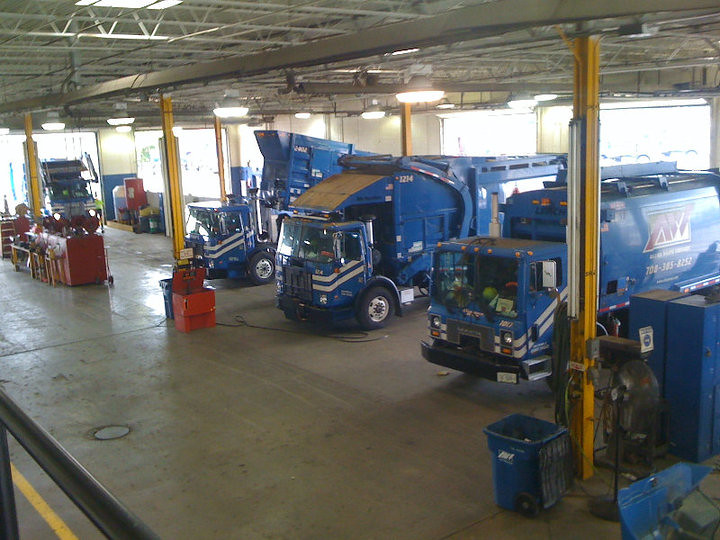The photograph depicts an expansive, hangar-like depot, designed for the storage and maintenance of sanitation trucks. The exceedingly tall ceiling, supported by metal and steel gantries, accommodates the trucks, some of which have their backs tipped at an angle, highlighting the vertical space available. Four large, bright blue sanitation trucks with diagonal white stripes on their cabs are parked inside the depot. These stripes vary in angle, adding a unique touch to each truck. 

On the right, one truck features a red logo or text, partially obscured, alongside a white phone number, faintly visible as 708-383-8252. The building's cement floor is demarcated by yellow posts, segregating the parking bays. Several large, red tool storage units are stationed at the back left, indicating a workshop area for vehicle maintenance. In the foreground, a blue wheeled trash bin with an indiscernible white textile logo and its lid removed sits prominently. The ceiling, adorned with lit rafters, and the presence of large garage doors underscore the functionality and scale of this depot, dedicated to housing and servicing these substantial blue trucks.